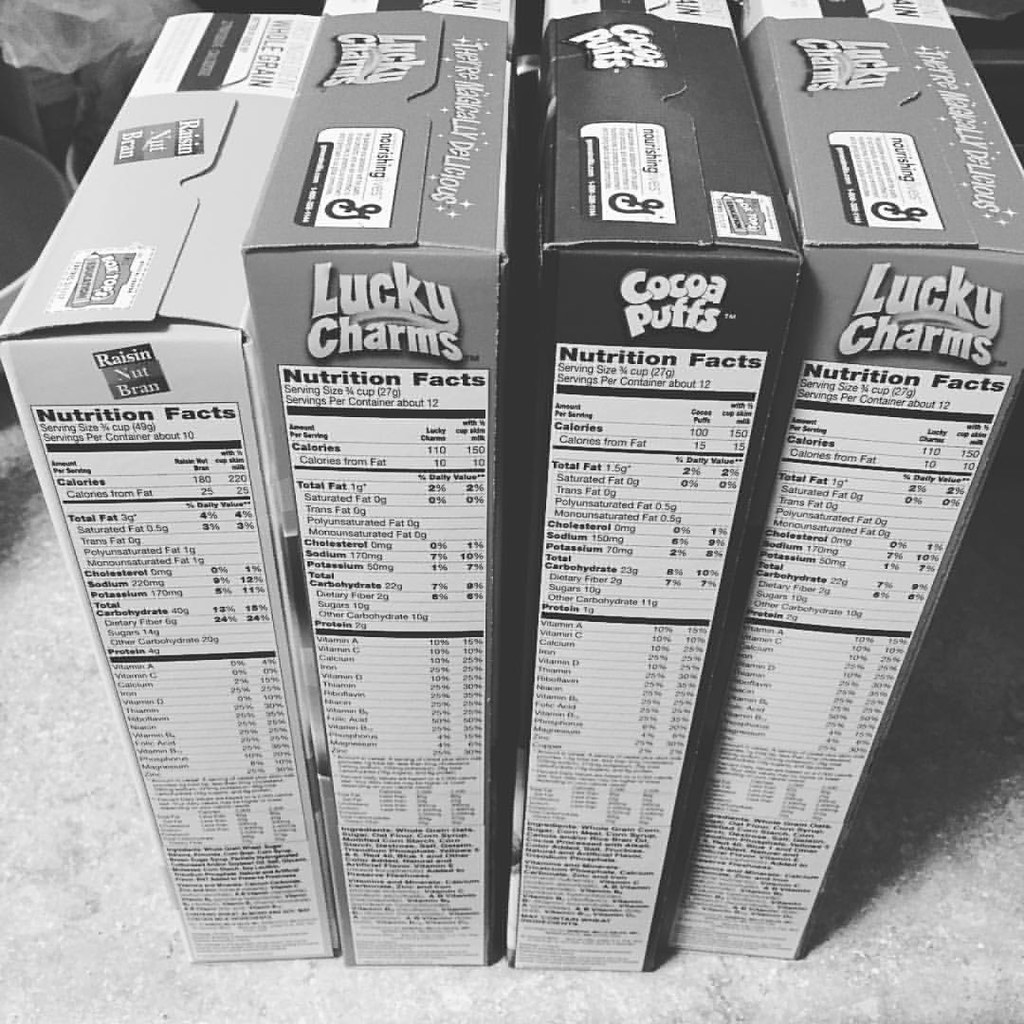This black-and-white photograph displays four unopened cereal boxes arranged side-by-side on a granite-like surface. The boxes are viewed from a slightly elevated angle, revealing both their nutrition facts labels and their tops. From left to right, the first box is Raisin Nut Bran, which features the Raisin Nut Bran logo and a Box Tops logo prominently on its front. Next to it is a box of Lucky Charms, followed by a box of Cocoa Puffs, and another box of Lucky Charms. All the cereal boxes are sealed, with their top flaps still glued together, indicating they have not been opened. This real-life image captures a neatly organized group of popular cereals, highlighted by the monochromatic color scheme.